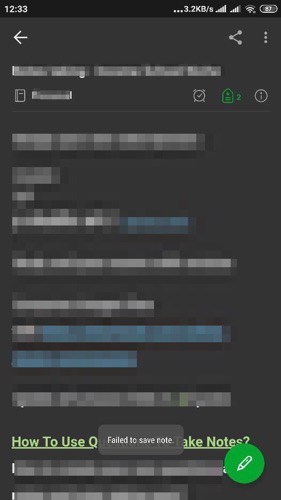Here is a cleaned-up and detailed descriptive caption for the image:

---

The image depicts a phone screen displaying a partially blurred interface. The top of the screen shows the time as 12:33 and indicates a data usage of 3.2 kilobytes, along with a strong reception signal. The main interface appears to be a note-taking application or perhaps QuickTime notes, with sections of the screen showing blurred content. In the center, there is a faint heading in light green text that reads, "How to use Q." Directly beneath this, a message notes, "Failed to save note." The interface features various text in gray and blue, with the blue text presumably clickable if it were not blurred. At the bottom of the screen, there is a green circular icon with a pencil, suggesting this button is for writing or editing notes. The overall screen background remains black, making the text stand out despite the blurring.

---

This caption retains all the critical details and organizes them into a coherent description.